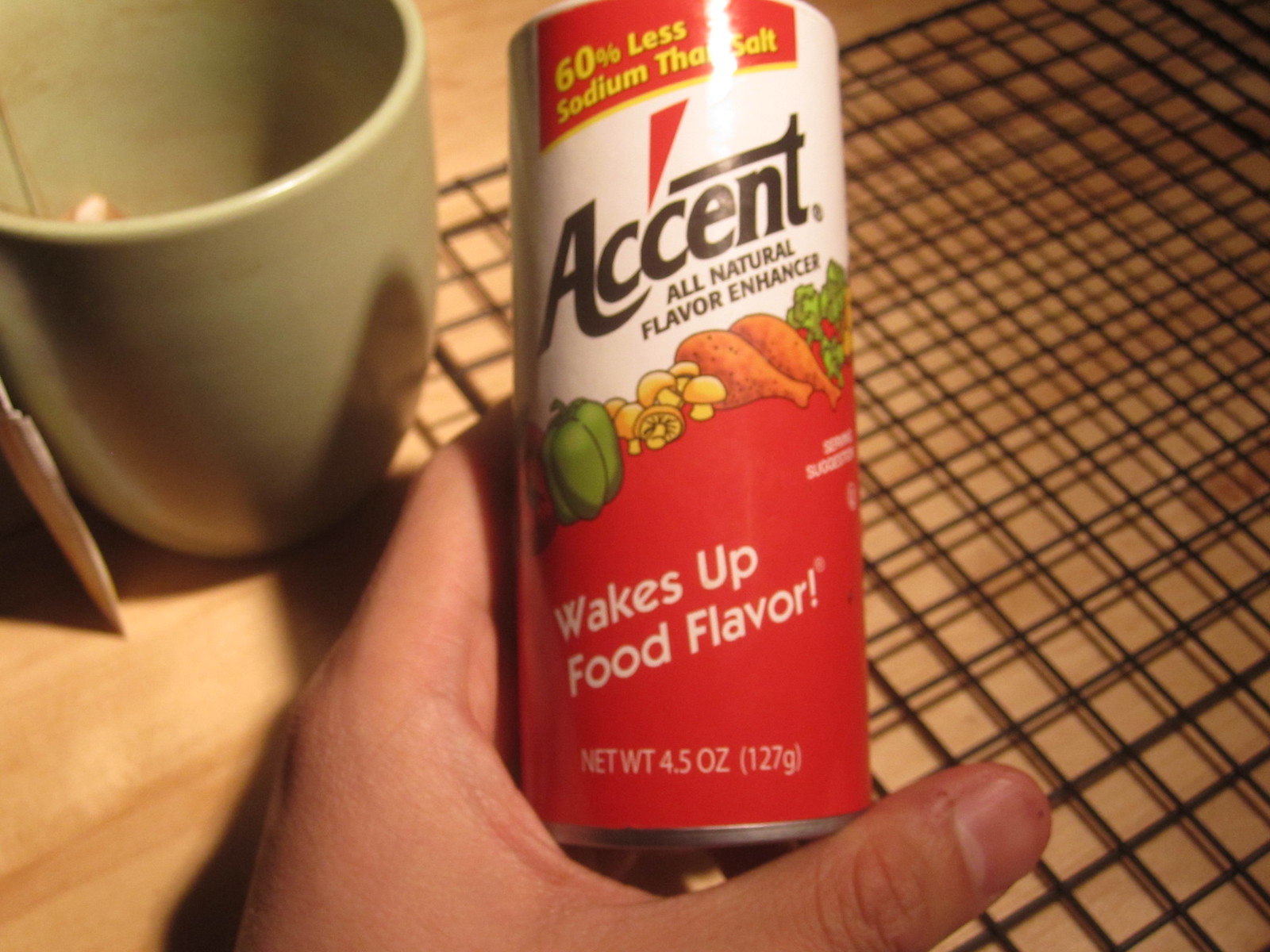A detailed photograph shows a white-skinned hand with a short thumbnail holding a small cylinder of Accent Flavor Enhancer. The can features a red and white label with various colored text and images. At the top, a red section with yellow text announces, "60% less sodium than salt." Below, on a white background, black text reads "Accent All Natural Flavor Enhancer," accompanied by illustrations of green bell peppers, mushrooms, chicken legs, salad greens, and possibly tomatoes or radishes. The lower part of the label has a red background with white text stating, "Wakes up food flavor" and the net weight, "4.5 ounces (127 grams)." The scene is set on a butcher block-style wooden table, with a black metal cooling rack in the background. To the left of the hand, a green mug with a teabag is visible, although the liquid inside is not discernible.